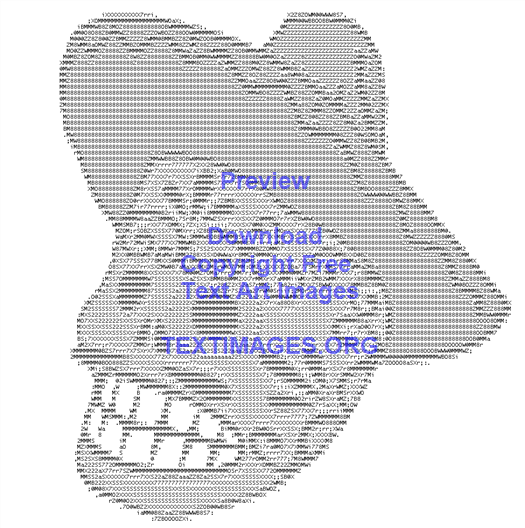The image showcases intricate ASCII art—a digital graphic formed through the arrangement of various computer text letters and characters. The backdrop is a clear white, providing a stark contrast to the design. Central to the piece is a detailed depiction of a skull facing left, its large white teeth prominently visible. The skull is adorned with a sombrero, a traditional wide-brimmed Mexican hat with a rounded crown. The skull features intricate designs, including leafy and floral patterns, with some motifs resembling a mustache carved into the structure. The entire image is monochromatic, rendered in shades of gray.

Superimposed on the skull, in blue, is text reading, "Preview. Download copyright-free text art images. Textimages.org." This watermark, positioned across the skull's face, underscores the image's availability on the mentioned website. Despite the lack of colorful decoration typically associated with similar Mexican-themed art, the image maintains a rich and detailed visual appeal through its precise use of typographic elements.